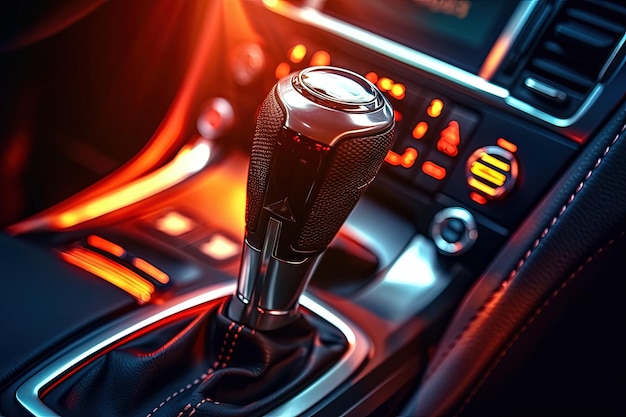The image depicts the luxurious interior of a car, focusing on the central console with particular emphasis on the gear shift. The gear shift is prominently silver and gray with a microphone-like appearance, positioned diagonally clockwise in the picture. Surrounding the gear, the console features an array of controls and buttons, illuminated in vibrant orange and yellow hues, suggesting a nighttime setting with the buttons and elements glowing softly. The dashboard reveals additional functionalities, including media player controls, air conditioning vents, and a variety of other buttons, all set against a dark leather finish with refined silver accents. To the right bottom corner of the image, there is black upholstery adorned with double rows of white stitching, enhancing the elegant design. The metal frame encircles the base of the gear shift, complementing the sophisticated aesthetic of the car's interior.